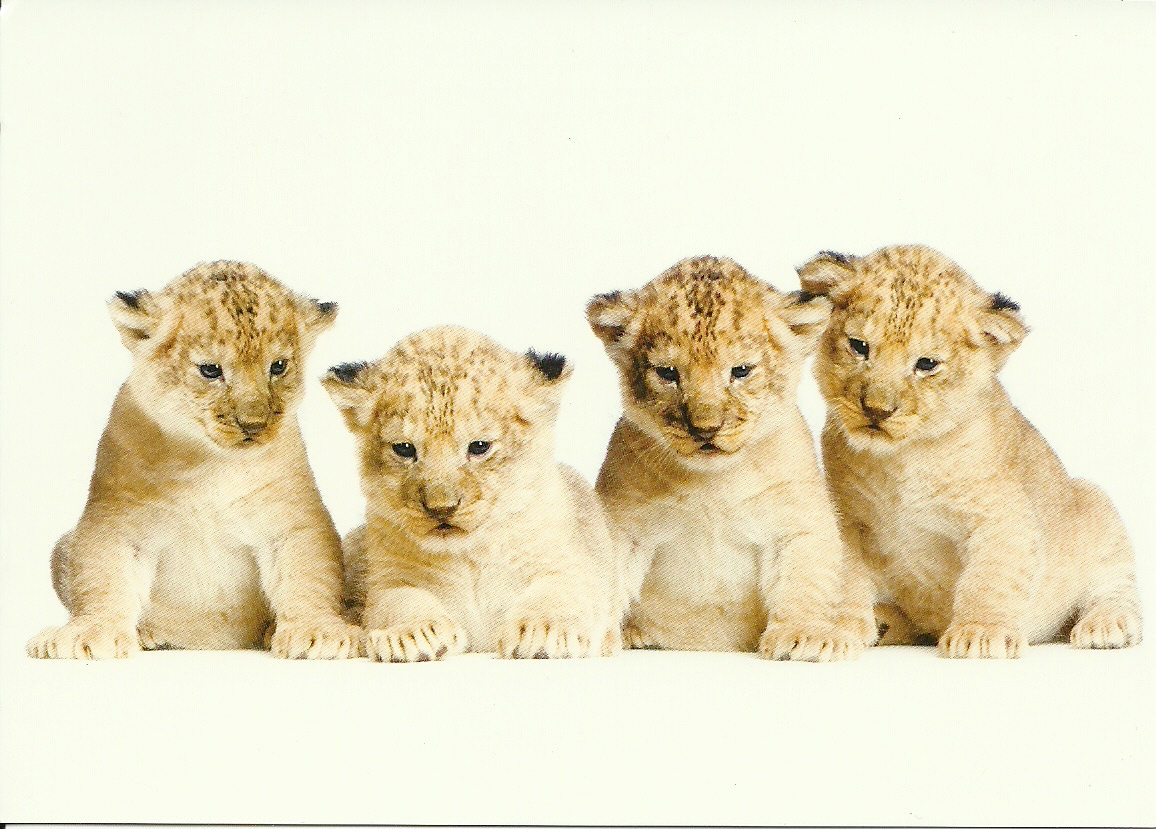This captivating image features four adorable lion cubs, aged around four to six months, perched on a seamless white counter or shelf that blends into the white background. The arrangement of the cubs begins with the leftmost one sitting upright, peering downward with an inquisitive gaze. Next to him, another cub lies down, extending its front paws while also looking over the edge. The third cub mirrors the posture of the first, sitting up but with one paw reaching behind the lying cub, and it too gazes downward intently. The final cub on the far right sits slightly angled inward, with its head cocked to the right as it also looks down below. These young cubs, with their light yellowish-brown fur adorned with dark brown spots and tufted ears, have an almost painted or drawn quality, accentuated by the serene, uniform background and surface. Their dark, expressive eyes and poised positions create a cohesive and touching moment captured in the photograph.